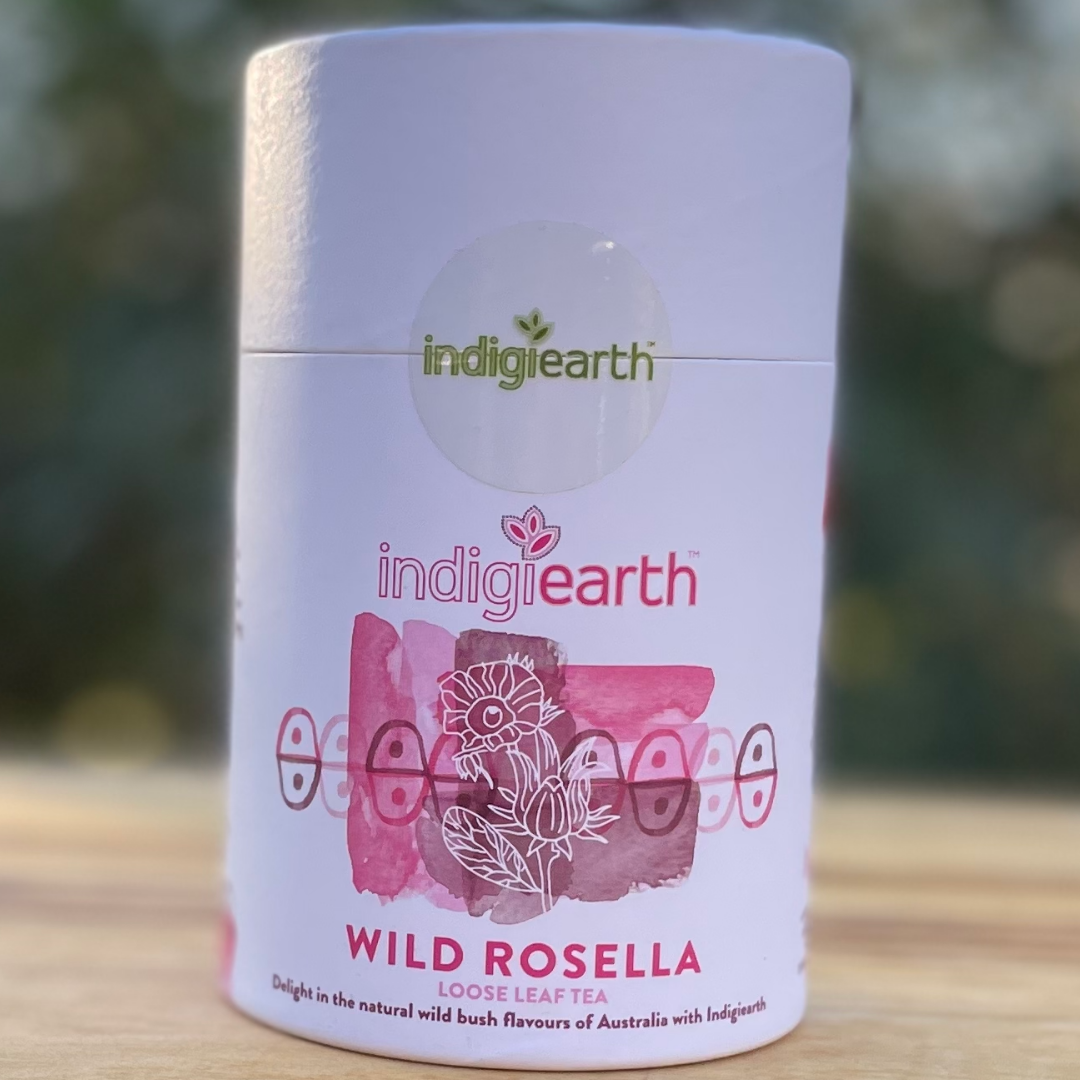This image is a close-up photograph of a white cylindrical container of loose leaf tea. The container has a detachable top section that separates from the bottom, with a clear round sticker bridging the seam between the two parts. This sticker reads "indigieearth" in green letters, with a small plant sprouting from the "I" to dot it.

On the front of the container, "indigieearth" is prominently displayed in white letters outlined in pink, and directly beneath is "earth" in pink letters. Below the text, there's an artistic image resembling a flower, composed of vertical and horizontal patterns in dark pink, light pink, and brown, interspersed with lines and half-circles containing dots. Additionally, a faint image of a plant is visible in the center of the design.

Further down, "Wild Rosella" is written in large pink letters, followed by "loose leaf tea" in fainter pink script. Another line of text in purple, partially visible above "Wild Rosella," reads "Delight in the natural wild bush flavors of Australia with indigieearth," though it is harder to discern in its entirety.

The overall aesthetic of the can is clean and detailed, with elements of both a minimalistic design and intricate floral artwork, reflecting the Australian wild bush theme.